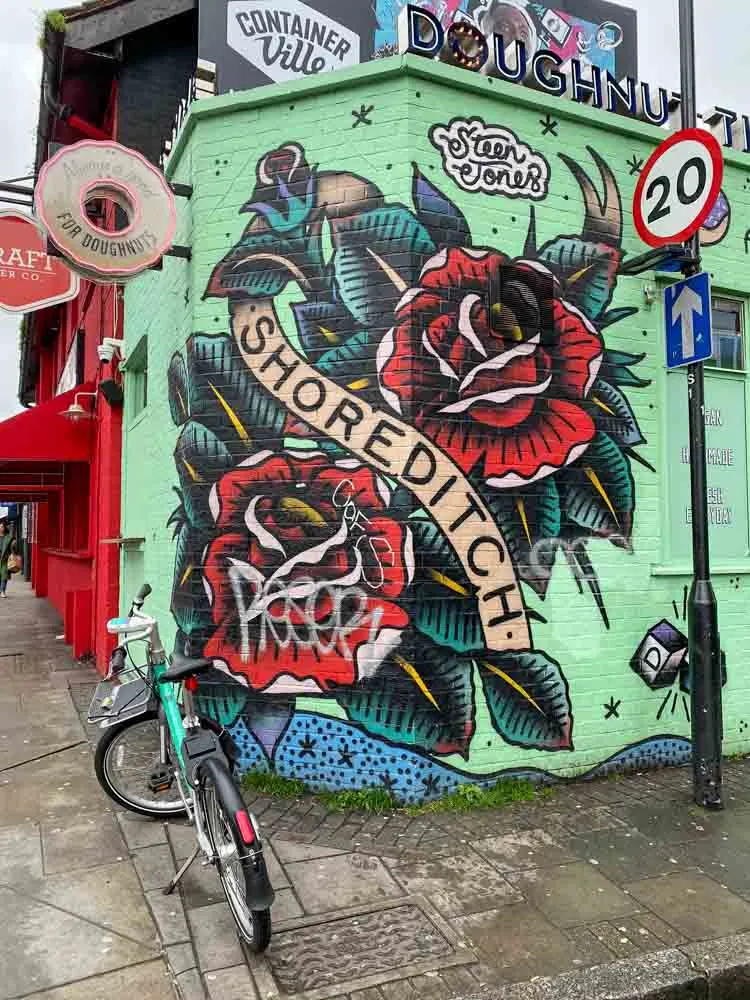This image depicts the side of a small brick building adorned with vibrant graffiti, viewed from the street. The building's wall, painted green, features a prominent mural that includes two striking red roses, one at the upper right and another at the lower left, surrounded by green leaves. Between the roses, the word "Shore Ditch" is artistically written. Additional graffiti includes the name "Steen Jones" and the letters "C.O.F.S." A signpost in front of the building bears two signs: one with the number 20 enclosed in a circle and another with a blue and white arrow. A teal and black bicycle is positioned on the stone sidewalk beside the building, suggesting a city environment. The image also reveals part of a red storefront which reads "4 Donuts and Craft Company" or possibly "Draft Company," and at the top, against a clear blue sky, there's writing that says "Don't Waste Time" and "Container Villa." Overall, the scene captures a colorful, urban streetscape with diverse elements of street art and local commerce.